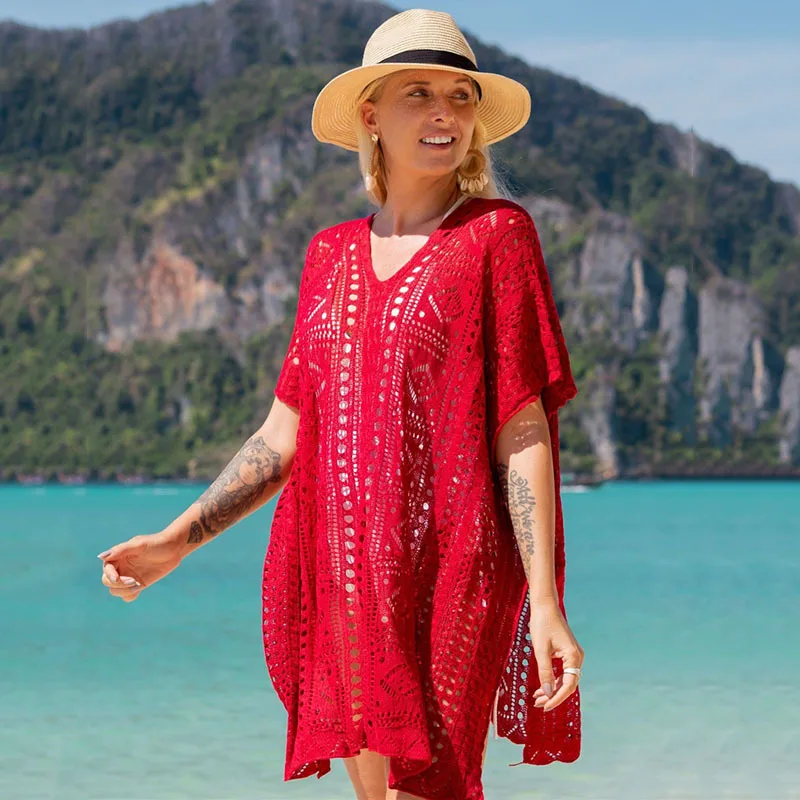In this vibrant photo, a woman of European descent stands smiling in front of crystal blue waters with a rugged, tree-covered mountain in the background. She is wearing a straw sun hat adorned with a black ribbon, and her blonde hair falls slightly above her shoulders. The woman is dressed in a lacy, crocheted red swimsuit cover-up, under which a white bathing suit is visible. The cover-up reaches just above her elbows, revealing large, intricate tattoos on both of her forearms—the one on her right arm is larger and darker, while the left arm features some writing. She also sports a ring on her right index finger and has shiny peach-colored skin. Adorning her ears are distinctive earrings; the right one is a long, circular piece with seashells hanging off the bottom, and the left earring features a large stone. Bare-legged, she is captured looking to the right, accentuating her bright smile and white teeth against the serene, teal-blue backdrop of water. The scene radiates tranquility, framed by clear, blue skies above the mountainous, tree-dotted terrain.